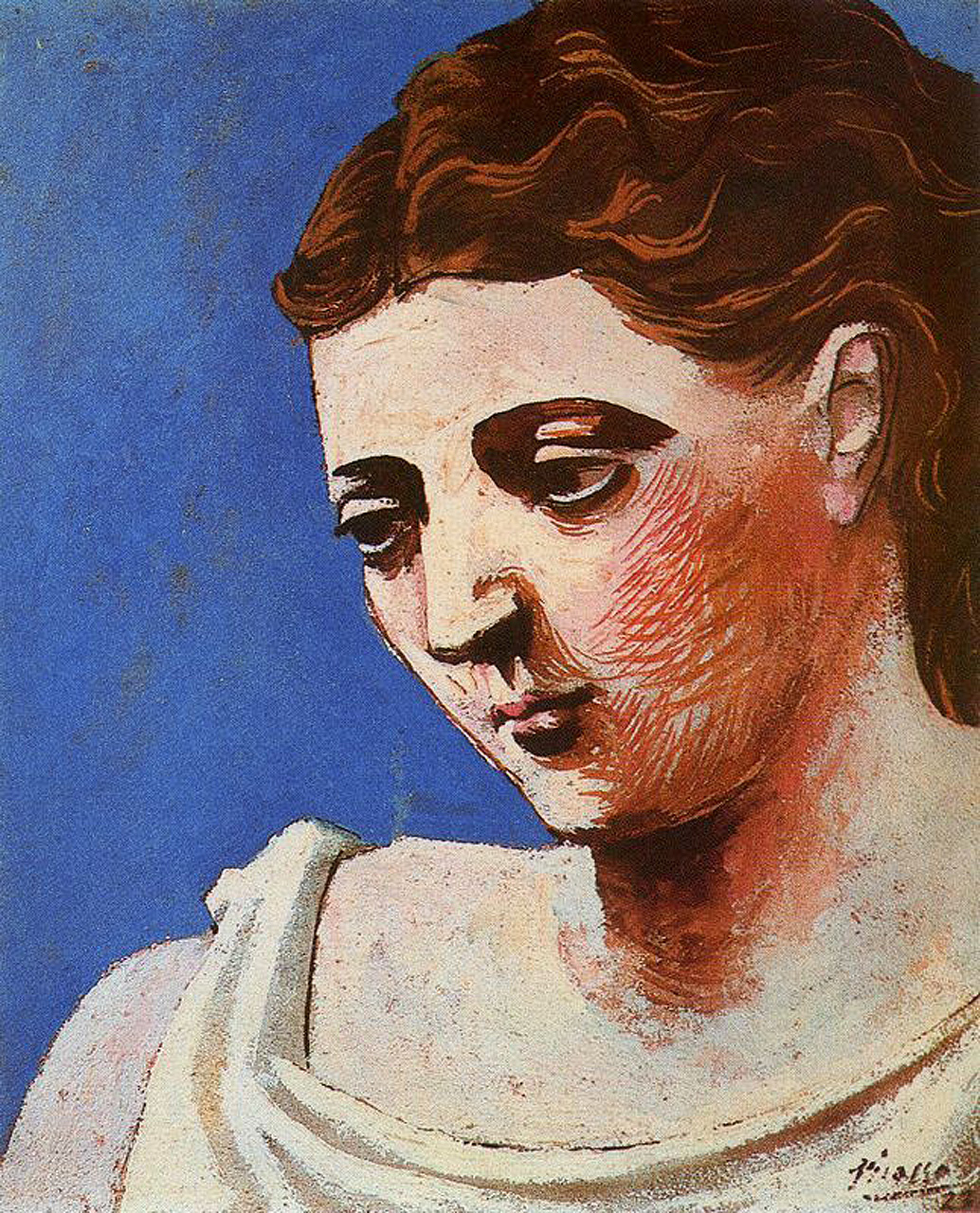This color painting, titled "Head of a Woman" and created by Pablo Picasso in 1923, is a portrait orientation abstract oil painting depicting a young woman with a refined Roman or Grecian influence. The background is a rich blue, accented with brown smudges and variations in color, particularly toward the upper left-hand corner. The woman, placed centrally but slightly to the right in the image, occupies the frame from just below her shoulders to the top of her head. She is angled such that her left side is nearer to the viewer, and her head slightly turned downwards, gazing towards the bottom left corner of the painting with a relaxed, possibly somber expression. 

Her dark red-brown hair is wavy, close to her scalp, and tucked behind her ear, revealing only her left ear. Her eyebrows are faint, barely more than straight lines leading into her heavy-lidded eyes. She has a prominent, straight nose and small, pouty lips. Her left cheek and neck are rendered with shades of red, giving her a flushed appearance. Donning a white garment reminiscent of a toga draped over her right shoulder, she exudes classical elegance. The painting is signed in the lower right-hand corner with what appears to be "MILSA 23."